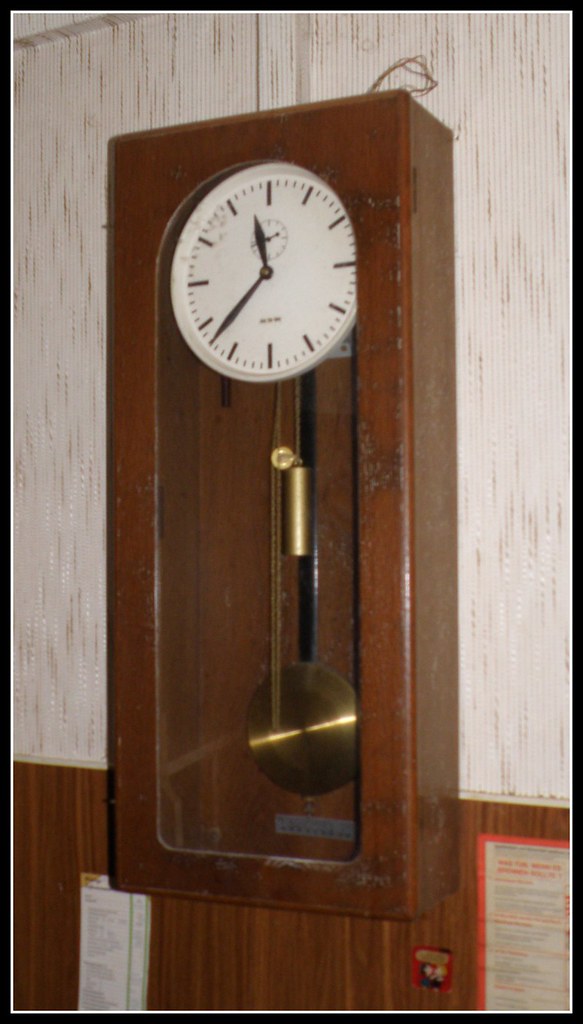The clock in the image is a distinctive, rectangular box-shaped timepiece, crafted from dark, almost reddish, wood. The front features a glass panel that reveals the clock's inner workings. The clock face, which is white and circular, is bordered by arched details at the top. Unlike traditional clocks, this one does not display numbers; instead, it has black tick marks to indicate the hours. The clock is equipped with black hour and minute hands, centered around what appears to be a gold-toned fastener. There is some text on the clock face, likely indicating the manufacturer's name, though it is not legible.

Beneath the clock face, a long, black metal rod holds a large, round pendulum that has a gold-toned or copper finish. Additional gold lines hang from the mechanism, one of which suspends another large, similarly gold-toned or copper-toned weight. The overall design and materials give the clock a vintage and elegant appearance.